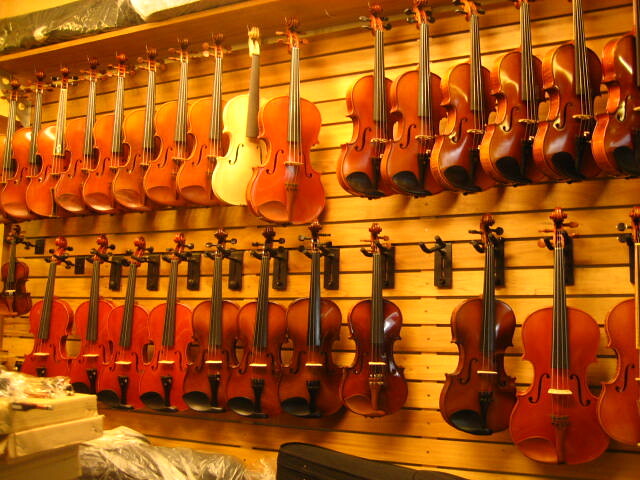This image captures a cozy, indoor scene of a stringed instrument music shop with soft yellow lighting. A wooden paneled wall serves as the perfect backdrop for showcasing a collection of violins and violas. There are two horizontal rows of instruments; the top row features 16 violins, including eight classic wood-colored violins with matching chin rests, one off-white violin, a viola, and six more violins with black chin rests, spaced slightly apart. The bottom row displays 12 instruments: four violins in lighter wood grain and three in darker wood grain with black chin rests, a smaller dark wood violin with a matching wood chin rest, another regular dark wood violin with a black chin rest, followed by a lighter wood viola, and another lighter wood violin. Some violins are held by their neck bows at a diagonal angle, while others are supported by their tuning pegs. Below the rows of violins, there are partial views of a fabric violin case, another case wrapped in plastic, and some stacks of boxes or trays. The arrangement and specific detailing, such as the mix of black and tan chin rests, suggest a specialized and carefully curated display, possibly indicating a violin repair shop or a specialized musical instrument store.